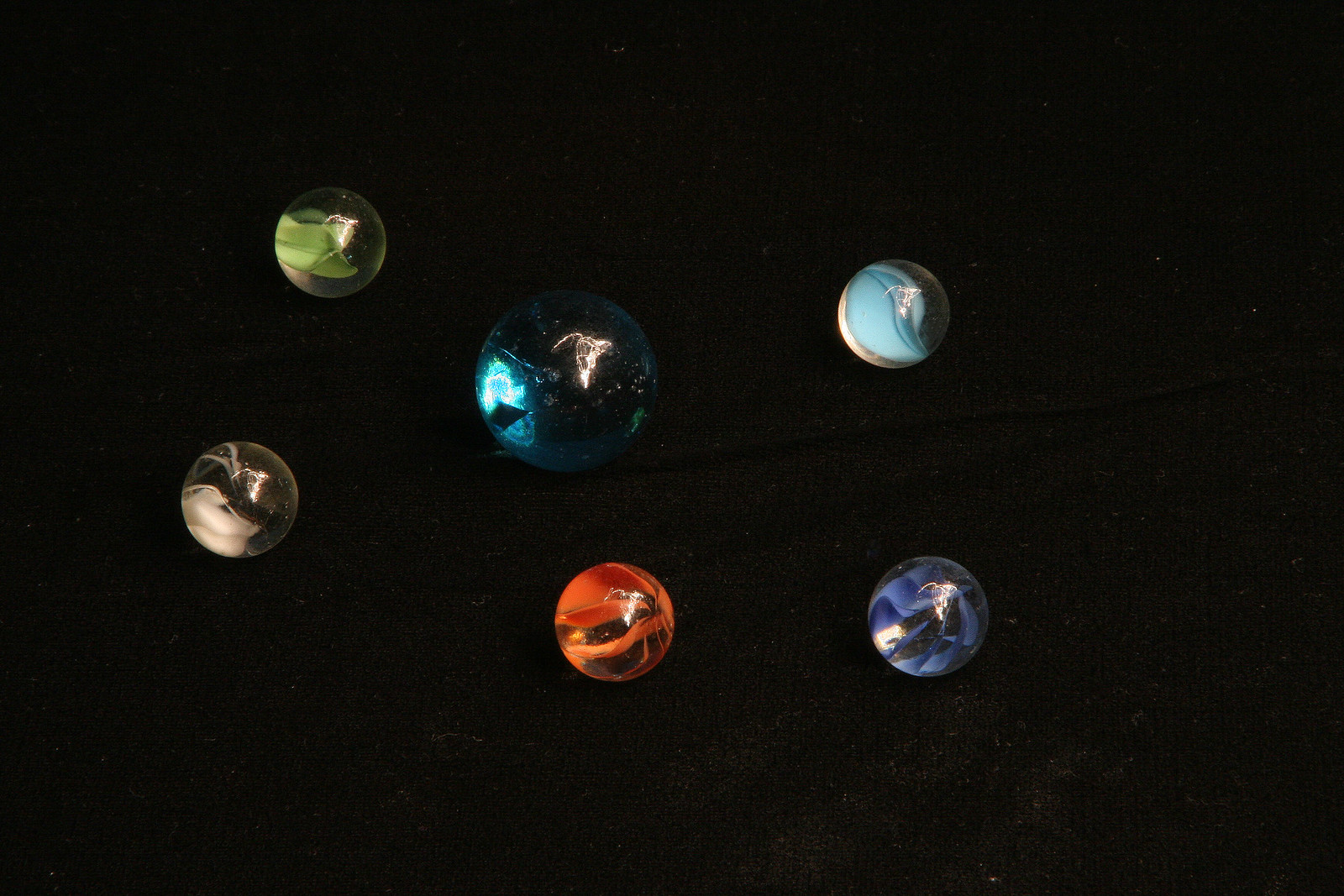This highly detailed, computer-generated image showcases six orbs set against a pitch-black background, reminiscent of the night sky but devoid of stars. The orbs are arranged in a celestial pattern, with the largest orb, a pearlescent blue, slightly to the left of the center. Surrounding it are five smaller orbs: a bright green one at the top left, a beige one just below it, a red-orange one directly beneath the large blue orb, a purple orb to the right of the red-orange one, and a blue and gold orb above the purple one. Each orb features intricate marbling, with the primary color intermixed with darker shades and reflective patterns that give them a glass-like appearance. The pattern on each orb resembles the shape of South America, mirrored horizontally, adding a unique, almost planetary yet surreal quality to the image.